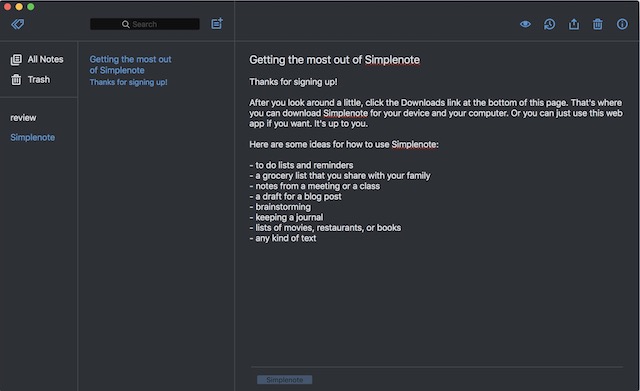The image depicts a macOS interface window with dimensions approximately one and a half times wider than it is tall, set against a dark gray background. In the upper left corner, the iconic red, yellow, and green traffic light buttons are clearly visible, indicating it is indeed a Mac machine. Directly below these buttons is a light blue icon resembling a tag.

Roughly 15-20% to the right of this tag icon is a black search bar, featuring a gray magnifying glass icon and the word "Search" in dimmed text, signaling users to input their queries. To the immediate right of the search bar, a light blue box with a plus sign sits in the upper right corner.

Further along, aligned to the far right, are five distinct icons, all in light blue. These icons include: an eyeball, a refresh symbol, a box with the left, bottom, and right walls intact and an arrow pointing upward from the top, a trash can, and a circle with an eye inside.

A horizontal gray line runs left to right, separating the bottom section of the window into three parts: approx. 10%, 20%, and 70% of the space, respectively. The leftmost segment appears to contain menu options, while the other sections are likely intended for additional content or features.